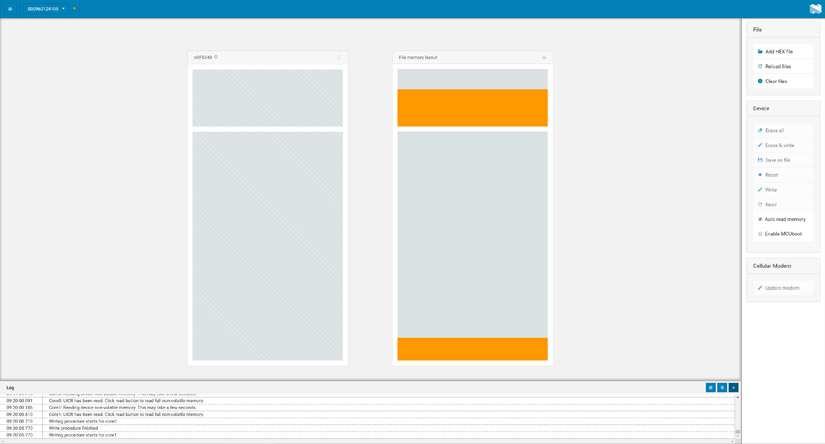Blurry image of a software interface, featuring a blue banner at the top. In the upper left corner, there's unreadable text, and a small symbol is situated in the top right corner. On the right side, there's a drop-down menu labeled "File," with three items beneath it, followed by another menu, possibly labeled "Device," and an option that reads "Cellular Modem." Below these options is a search icon that resembles a pencil. The main area of the interface displays a blank grayish-white screen with two central rectangular boxes. The first box is white with a gray border, consisting of a smaller rectangle at the top and a larger one at the bottom. The second rectangular box has a gray background with orange splotches at the top and bottom, resembling an editable template for design work. At the bottom of the interface, there's a section labeled "Log," featuring dates on the left side and a note-taking area on the right side, likely intended for personal notes within the software. Though the details are indistinct due to the blurriness, the structure suggests an editable workspace with logging capabilities.